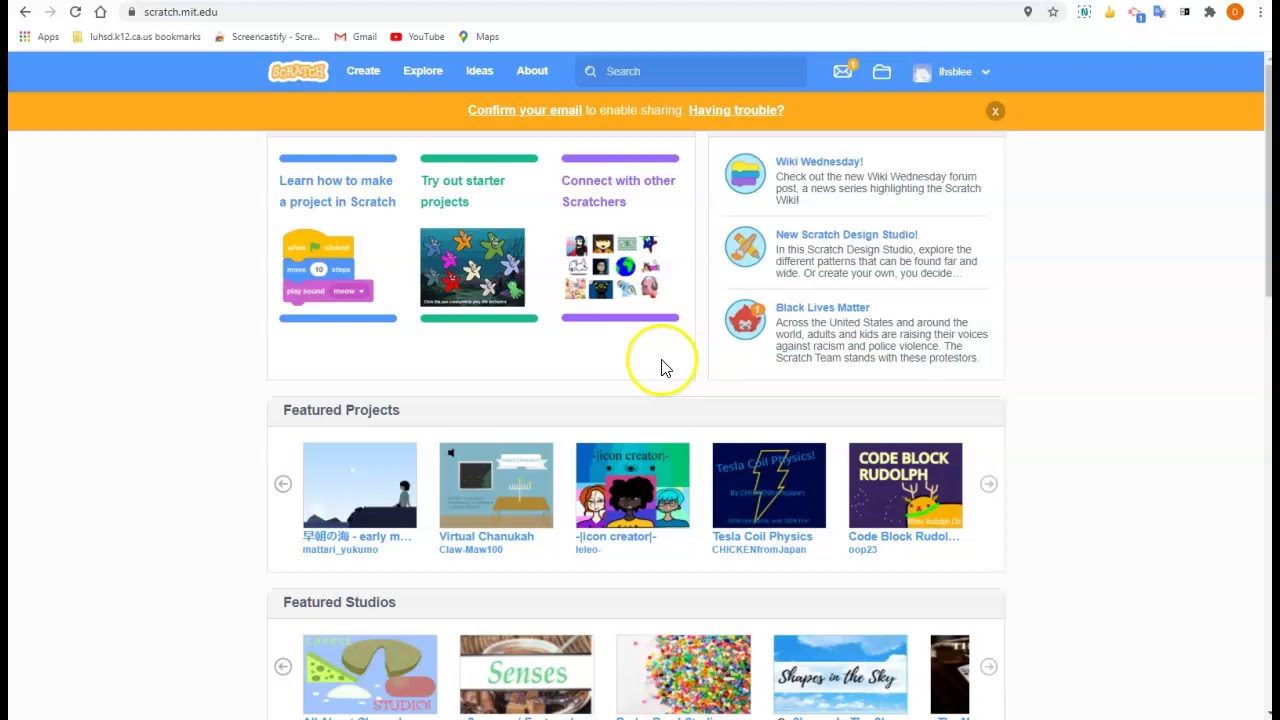This image is a detailed screenshot of a website viewed in a Windows browser. The browser's address bar prominently displays the URL "grass.mit.edu," and underneath it, several bookmarked items are visible, including "Apps," a brown folder whose label is difficult to read, "Screencastify," "Gmail," "YouTube," and "Maps."

The website's layout is centered on the screen, featuring a light blue border at the top that houses the main navigation menu. On the left side of the border is the Scratch logo, designed in yellow bubble letters. The navigation menu includes links labeled "Create," "Explore," "Ideas," and "About," all written in white letters. To the right, there's a search box with a magnifying glass icon and the word "Search" in white. Further right are icons for notifications, folders, an avatar, a small, indistinguishable username, and a dropdown caret.

Below the blue border, a thin, rectangular yellow-orange notification bar spans the width of the page. It reads, "Confirm your email to enable sharing," with the phrases "Confirm your email" and "Having Trouble?" both bolded and underlined.

The main content area of the website has a white background and is divided into several sections. The top section on the left contains three blocks with images:
1. A block with a thin blue border, featuring the text "Learn how to make a project in Scratch," accompanied by smaller, colored rectangular boxes.
2. A green-bordered block with the text "Try Out Starter Projects" and an image of a cartoonish underwater scene with various starfish.
3. A purple-bordered block labeled "Connect with Other Scratchers," showcasing a line of cartoon avatars.

To the right of these blocks is another rectangular section with three linked images:
1. An image with yellow, green, and fuchsia rectangles and the text "Wiki Wednesday" in blue, followed by the description "Check Out the New Wiki Wednesday Forum Post."
2. An image of a blue circle with a paintbrush and pencil crossed, accompanied by "New Scratch Design Studio" and a description encouraging creative pattern exploration.
3. An image of a cartoon monkey head within a blue circle, paired with "Black Lives Matter" and a supportive message from the Scratch Team.

Further down, two larger rectangular boxes with gray headings are displayed:
1. "Featured Projects," showcasing five thumbnail images labeled "Some Foreign Writing Early," "Virtual Hanukkah," "Icon Creator," "Tesla Coil Physics," and "Cold Black Rudolph."
2. "Featured Studios," featuring five more thumbnail images with cartoonish depictions of candy, the sky, and various foods. Some names are cut off, requiring scrolling to view fully.